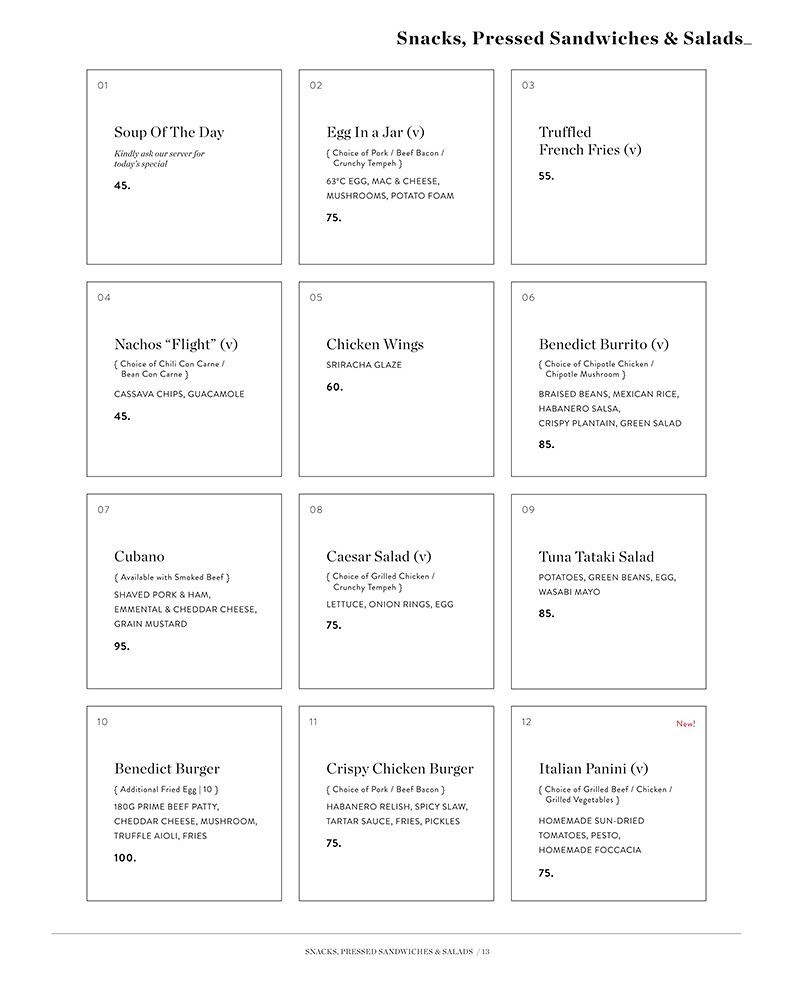The image displays a portrait-oriented menu titled "Snacks, Pressed Sandwiches, and Salads" at the top in bold black text. The menu is structured into 12 numbered squares arranged in three columns and four rows. Each square contains the name of a dish, a price number, and occasionally a brief description of ingredients. The numbering begins from the top left and proceeds left to right and top to bottom, numbering each item from 1 to 12.

1. **Soup of the Day** - 45
2. **Egg in a Jar** - 75
3. **Truffle French Fries** - 55
4. **Nachos Flight** - 45
5. **Chicken Wings** - 60
6. **Benedict Burrito** - 85
7. **Cubano** - 95
8. **Caesar Salad** - 75
9. **Tuna Tataki Salad** - 85
10. **Benedict Burger** - 100
11. **Crispy Chicken Burger** - 75
12. **Italian Panini** - 75

Most squares feature brief descriptions beneath the dish names, detailing the ingredients. The menu uses a simple black-and-white design, focusing on clarity and organization.